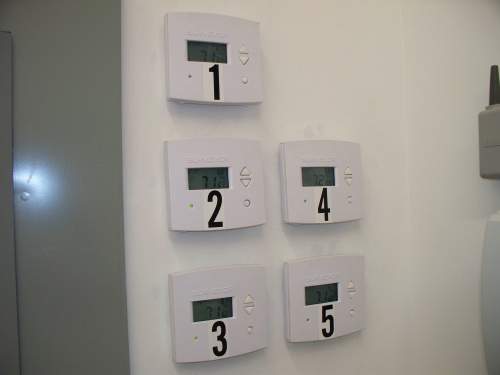This photograph captures a neatly arranged set of thermostats mounted on a pristine white wall. The thermostats are ordered and numbered with three in a vertical column on the left labeled 1, 2, and 3 from top to bottom. To the right of this column are two additional thermostats, numbered 4 and 5, aligned vertically and matching the height of the lower two on the left.

The image is primarily head-on but taken from a slightly leftward angle. The white wall behind the thermostats is immaculate, enhancing the clean presentation of the scene. To the left edge of the photo, part of a gray metal panel, likely the edge of a door frame, is visible. This panel includes a single screw midway up with subtle light reflections indicating minor warping around the screw.

Two other objects are partially visible on the right side of the frame, with one white and tall at the bottom, and a shorter gray object at the top, though not enough is visible to identify these items. 

Each thermostat is a white rectangular unit featuring a gray display screen toward the left side, showing the current temperature setting. On the left side of each display, large black numbers clearly indicate the temperature: thermostats 1, 2, 3, and 5 are set to 71°F, while thermostat 4 is set to 72°F. The controls on the thermostats consist of an up arrow, a down arrow, and a circular button positioned on the right side, providing a straightforward interface for adjustments.